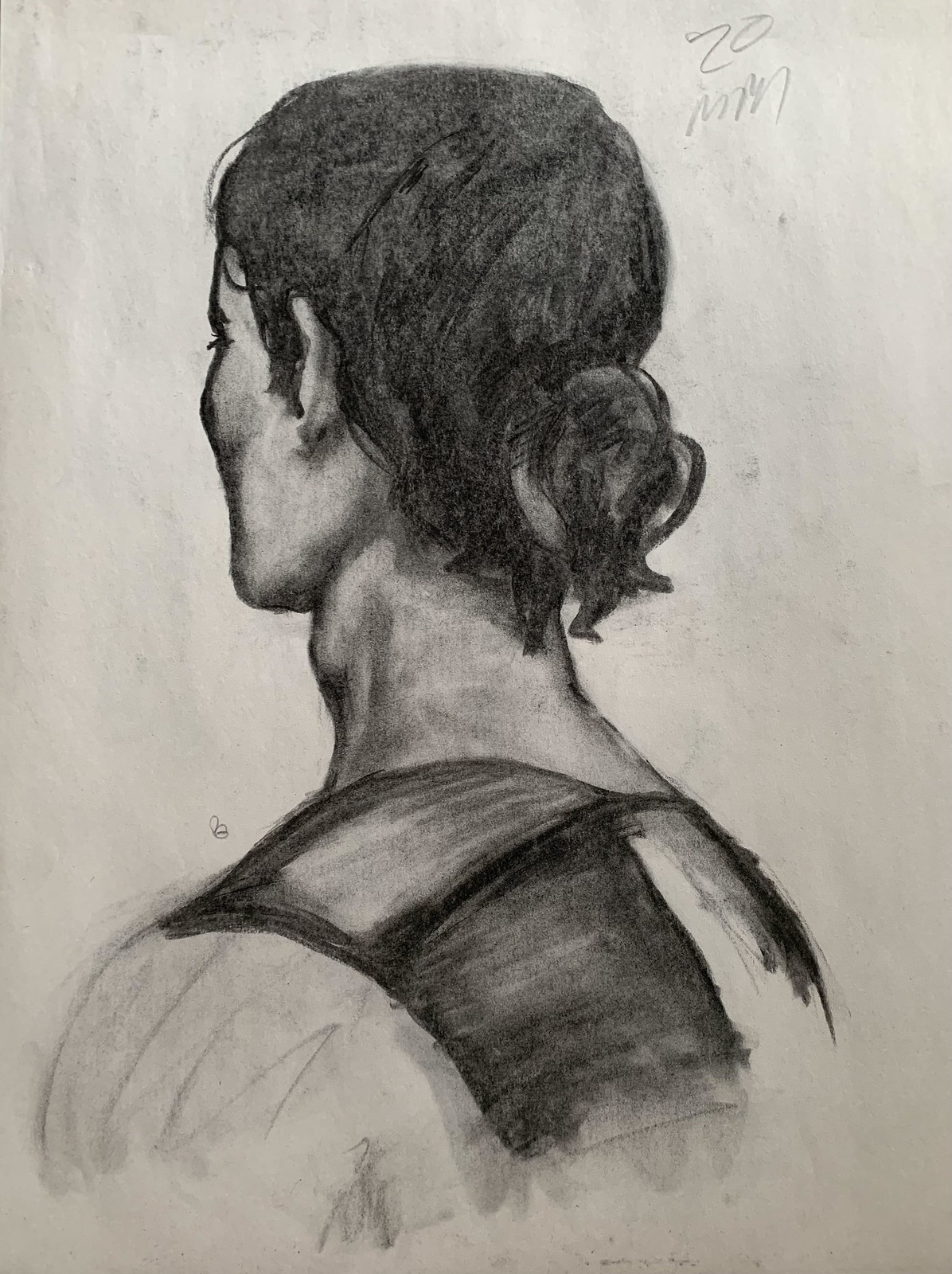This hand-drawn pencil sketch is an artist's rendering on white paper, showcasing a person from behind. The overall shape of the image is rectangular, with the longer sides on the left and right. In the center, the person is depicted with their back and left shoulder visible, their dark hair pulled back into a loose bun at the nape of their neck. The figure has broad shoulders and a defined side cheek, with an ear slightly visible. The attire appears to be a vest with an open back or a tunic, marked by shaded squiggled pencil marks on the sleeve. The white paper has various dark smudges, perhaps from the drawing process. In the top right corner, the sketch is signed with what appears to be '20MM' or 'ZO-MM'. The detailed shading and perspective give the drawing an evocative and intimate feel.